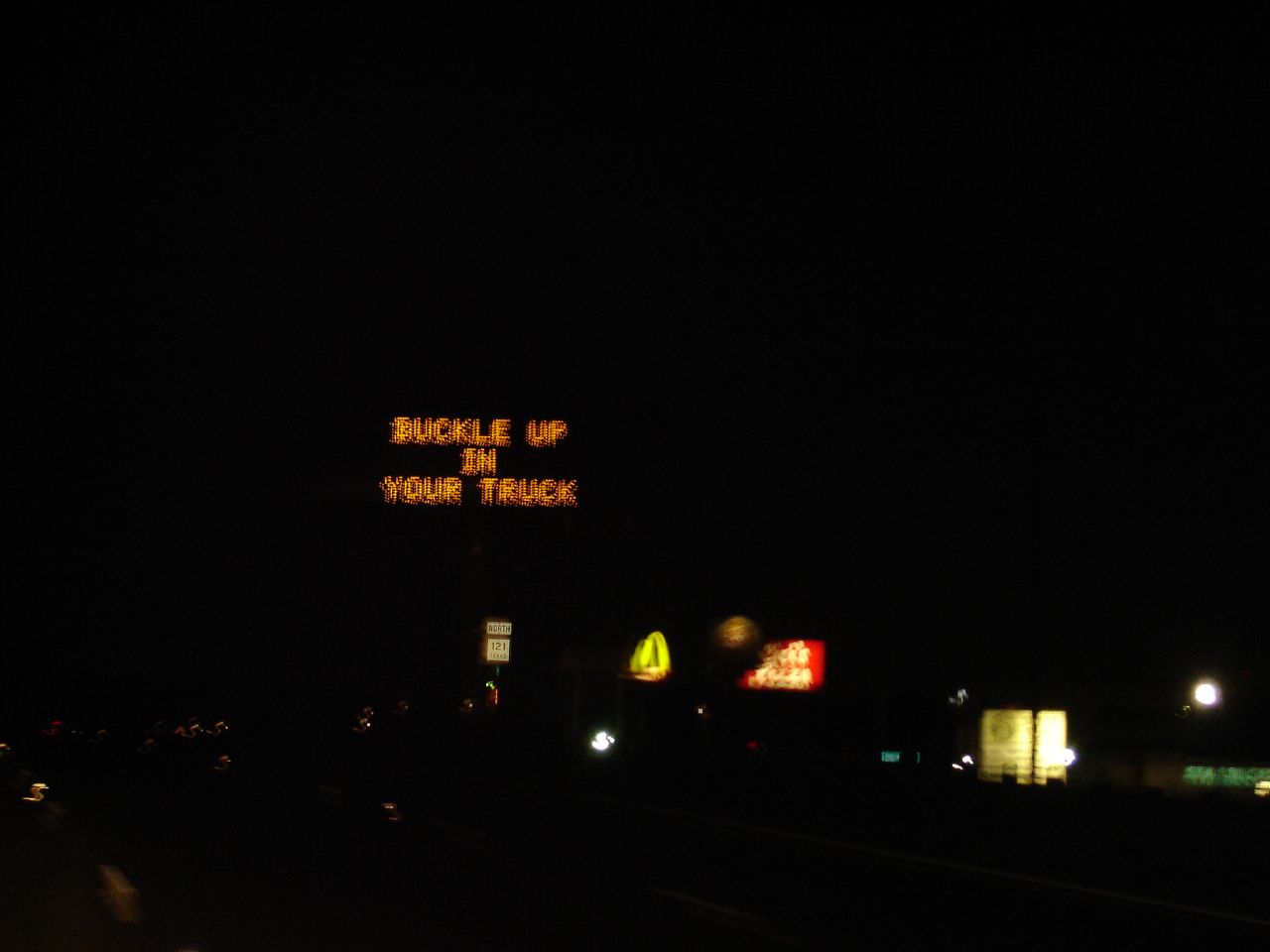In this nighttime photograph, minimal lighting casts a dim ambiance over the scene. The focal point is a large, illuminated sign elevated approximately 30 to 40 feet above the ground. This sign, constructed from individual LED lamps, clearly displays the words "Buckle Up In Your Truck." Below this prominent sign, several smaller signs are visible, though their text is indiscernible from the current perspective. The scene also includes a building to the right, distinguishable by a light that highlights its yellow exterior wall. The photo captures a roadway, evident by the faint visibility of yellow lines that mark the lanes, adding depth and context to the nocturnal landscape.